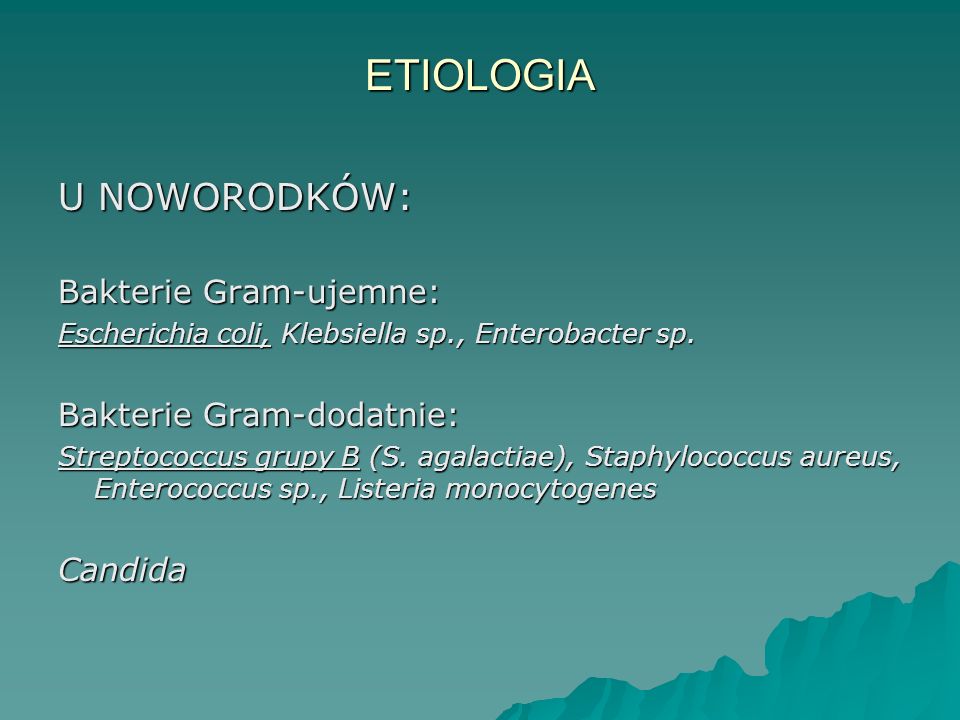The image appears to be a computer screenshot of a PowerPoint presentation slide, primarily formatted in aqua blue with varying shades of blue used throughout. The focal point of the slide is the title "ETIOLOGIA" written in large, yellow text at the top center. The slide features multiple lines of white text, listing terms, presumably related to biology or microbiology, such as "Bacterigram," "Staphylococcus aureus," "Streptococcus group B," and "Candida." The layout suggests it's part of a more extensive presentation. In the lower right corner, there is a design element resembling rock formations or a mountain range, also in an aqua blue hue. The slide is slightly wider than it is tall, and overall, it showcases a well-structured format with a clear emphasis on etiological terminology.